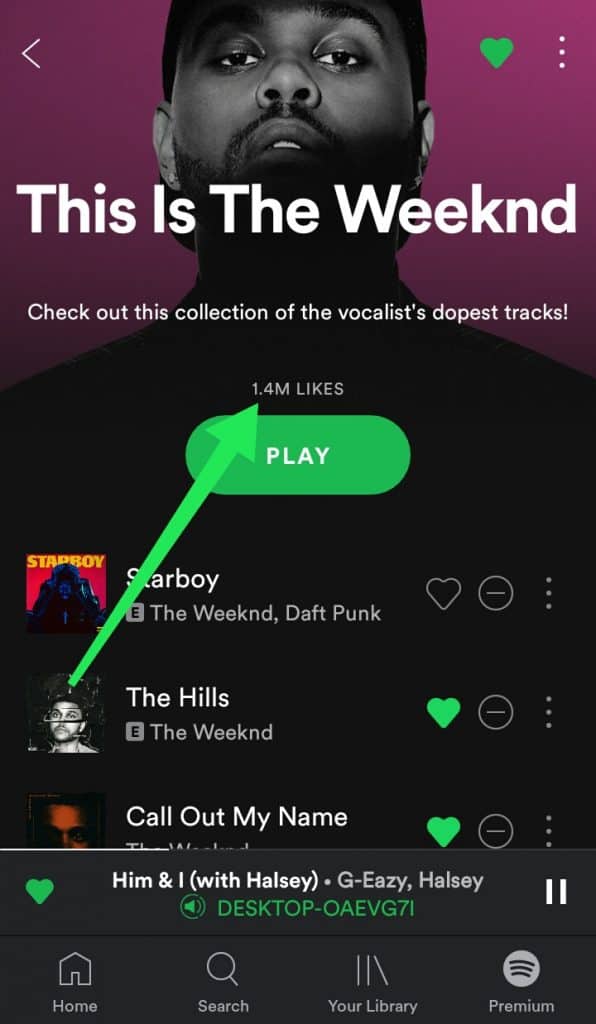Screenshot of a smartphone displaying a music app interface featuring The Weeknd:

The image showcases a black-and-white photograph of an African-American man with a mustache, presumably The Weeknd. He appears somber, with his head slightly tilted down and a partial view of his teeth. The photo gradually fades into black below his bottom lip, revealing the silhouette of his neck and shoulders against a purple background.

To the left of the head is a white arrow icon pointing left, while to the right are a green heart icon and a vertical ellipsis (three dots). Below these icons, the text "THE WEEKND" is displayed in white uppercase letters, with "WEEKND" notably spelled without the 'E'. Further below, in smaller white text, it reads: "Check out this collection of the vocalist's dopest tracks!"

Beneath this description, there is a statistic showing "1.4M LIKES" in white text. An oval green button with the word "PLAY" in all caps occupies the center below the likes, and a green arrow points from "1.4M LIKES" down to the second icon on the left-hand column of the app.

On the left side of the screen, there are three user response icons. The first icon features a colorful album cover with "Starboy" written in yellow on top of a red and black background. Next to it, in white text, is "Starboy" again with a gray box below containing a black letter "E" and the text "The Weeknd - Daft Punk" (TWDP). The following icons include a gray heart, a gray circle with a white minus sign, and vertical gray dots.

The second image, pointed to by the green arrow, is a black-and-white image of another person, presumably another user. It features the name in all caps: "TAT HILLS". Below it is another gray box with the letter "E" and "TWNED" with a heart icon next to it.

The third image shows another person’s eyes and eyebrows in a slightly reddish hue. Next to the image, in capital letters, it says "Call Out My Name" with similar icons: a green heart and a white circle with a horizontal line.

Across the bottom of the screen, there's a menu with four icons: a house labeled "Home", a magnifying glass labeled "Search", a book icon labeled "Your Library", and a circular icon with three lines labeled "Premium".